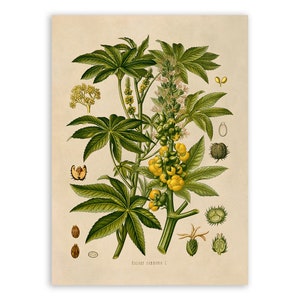The image depicts a vertically oriented, detailed illustration of various plants on a rectangular sheet of beige-colored paper which casts a slight drop shadow against a white background. The central focus of the drawing features two prominent green stalks adorned with long, verdant leaves sprouting outward. These stalks support small yellow fruits or fluffy flowers that resemble either mini lemons or cauliflower buds. Surrounding the main plants are additional detailed drawings of seeds and nuts, including small brown circular seeds and dark nuts. The illustration exhibits a hand-painted or hand-drawn style, though it might be computer-generated to mimic such an effect. Black text is present at the bottom of the image but is not legible. Overall, the composition balances the central stalks with additional botanical details, providing a rich, comprehensive depiction of the plant life.